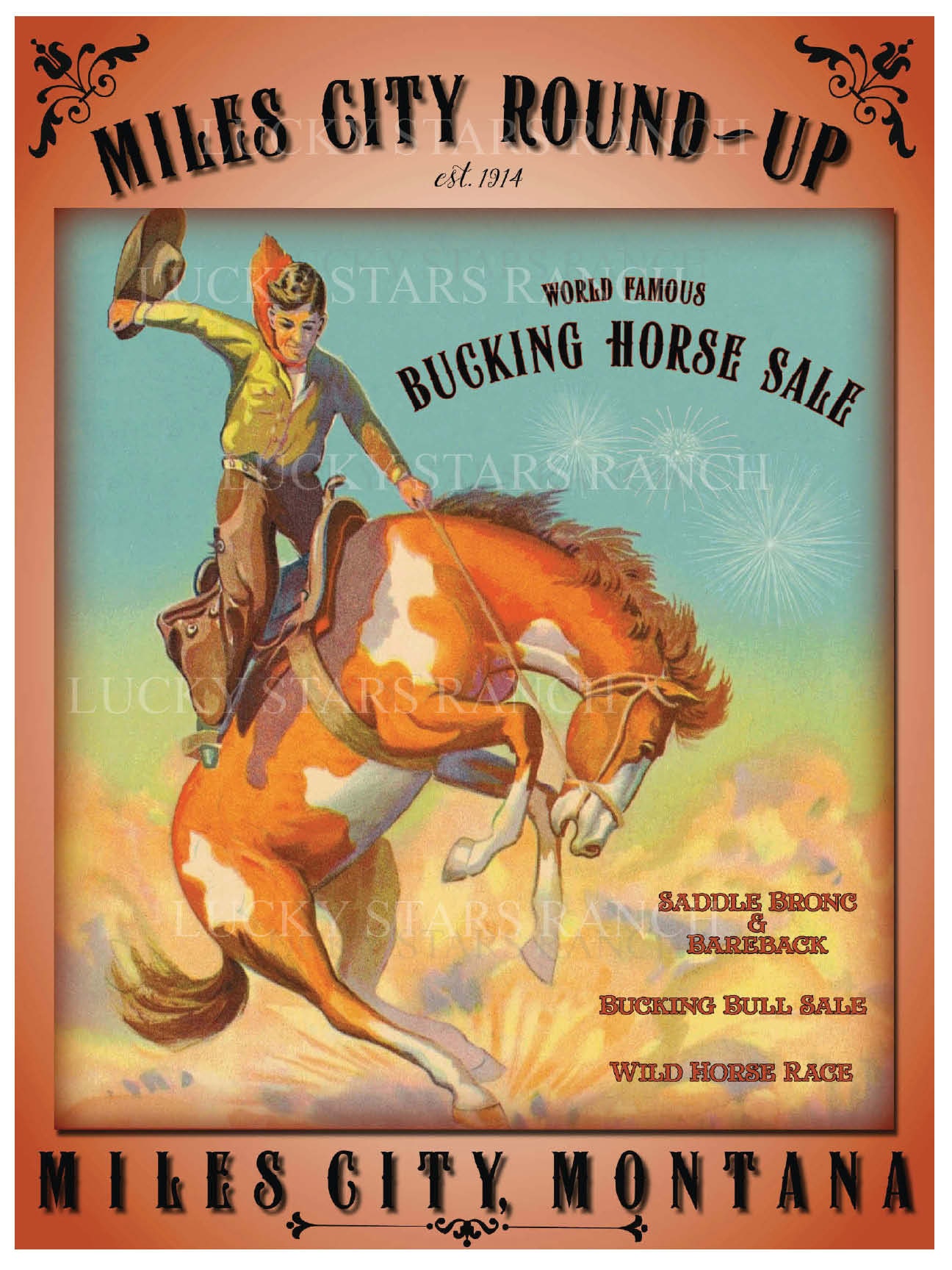The image, resembling a front cover of a magazine or a poster, features a vibrant orange border that transitions into a lighter orange gradient at the center. At the top, the text "Miles City Roundup" arcs in black letters, with "EST 1914" directly below it. The decorative elements in black adorn the upper corners. A prominent illustration captures a dynamic scene: a young boy, dressed in a green shirt and brown chaps, rides a brown and white bucking horse rearing on its hind legs. The boy brandishes a cowboy hat in one hand and grips the reins with the other. The text "World Famous Bucking Horse Sale" is positioned in the upper right corner of the illustration. Additional text in the lower right reads, "Saddle Bronc and Bareback Bucking Bull Sale, Wild Horse Race." Watermarks bearing the name "Lucky Stars Ranch" overlay the image. Finally, "Miles City, Montana" is printed at the bottom of the poster.